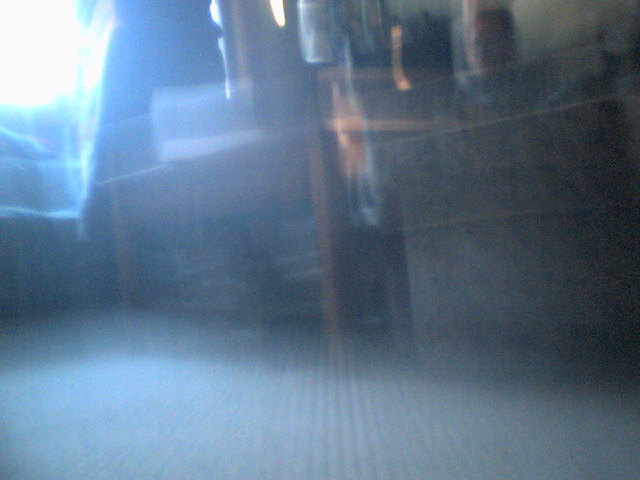This landscape-oriented image is distinctly blurry, obscuring any definitive identification of its contents. The composition features a downward-sloping floor starting from the left, creating an angled perspective towards the right. In the upper left-hand corner, a bright white light source, surrounded by a blue halo, emits rectangular-shaped afterimages, drawing the viewer's focus. On the left side of the image, there is a faint outline of what might be a desk, surrounded by miscellaneous objects scattered toward the back and right side, all situated at varying levels. The overall color palette is muted with low saturation and brightness, except for the intense luminosity from the light source, suggesting the photograph might either be AI-generated, highly out of focus, or taken with the camera in motion.